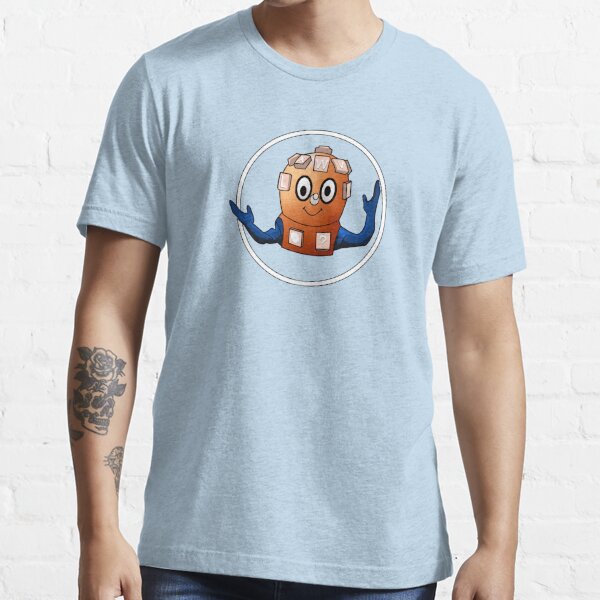This is an image of a light blue, crew neck t-shirt worn by a male model standing against a bright, white-painted brick wall. The photograph captures the man from just below his chin to just below his waist, showing his torso prominently. The t-shirt features a distinct design at the center: a white circular border enclosing a brown, robotic creature with big white eyes that have black dots in the middle. The creature has squares resembling computer keyboard keys on top of its head and chest. It sports a black smiling face and extended blue arms, with the right hand facing upwards and the left hand pointing upwards and slightly to the left. The man's arms hang straight down, revealing detailed black tattoos, including a skull topped by a flower with vines extending through its eyes and other openings. The overall scene exudes a bright and airy atmosphere.